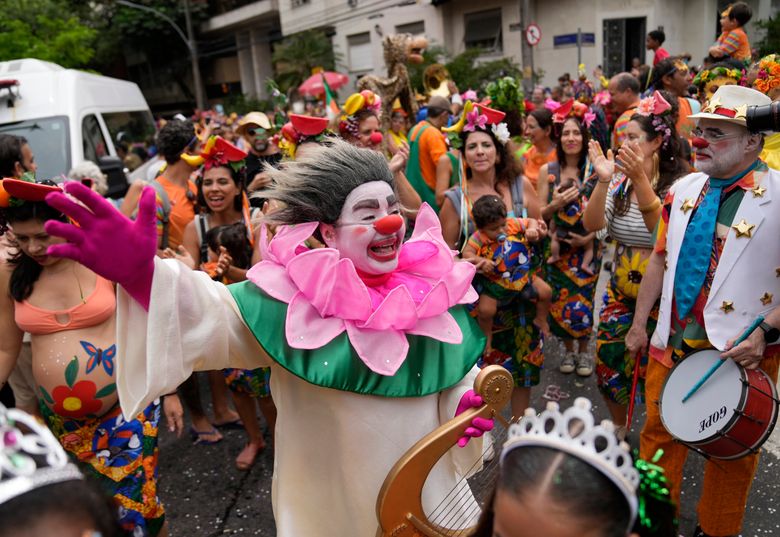In this vibrant photograph captured from the heart of a bustling parade, the central figure is a cheerful clown, distinguishing the scene with his exuberant presence. The clown dons a distinctive red nose and a striking gray wig styled to stick straight up, reminiscent of Don King's iconic hair. His outfit is elaborate, featuring a large collar composed of three layers—pink, lighter pink, and green—resembling the petals of a flower. He wears pink gloves and a flowing white robe. With a broad smile, he waves enthusiastically at the crowd.

To his right, another clown, similarly adorned with a red nose and dressed in a white jacket, stands merrily with a drum set. On the clown's left, a woman who appears to be pregnant joyfully displays her belly, painted with vibrant flowers. The background is filled with a diverse group of people clad in brightly colored clothing and hats, adding to the festive atmosphere. Behind this lively assembly, residential houses are visible, indicating the parade is taking place in a neighborhood street. The scene is a vivid tapestry of colors and joyous celebration, capturing the essence of community and festivity.